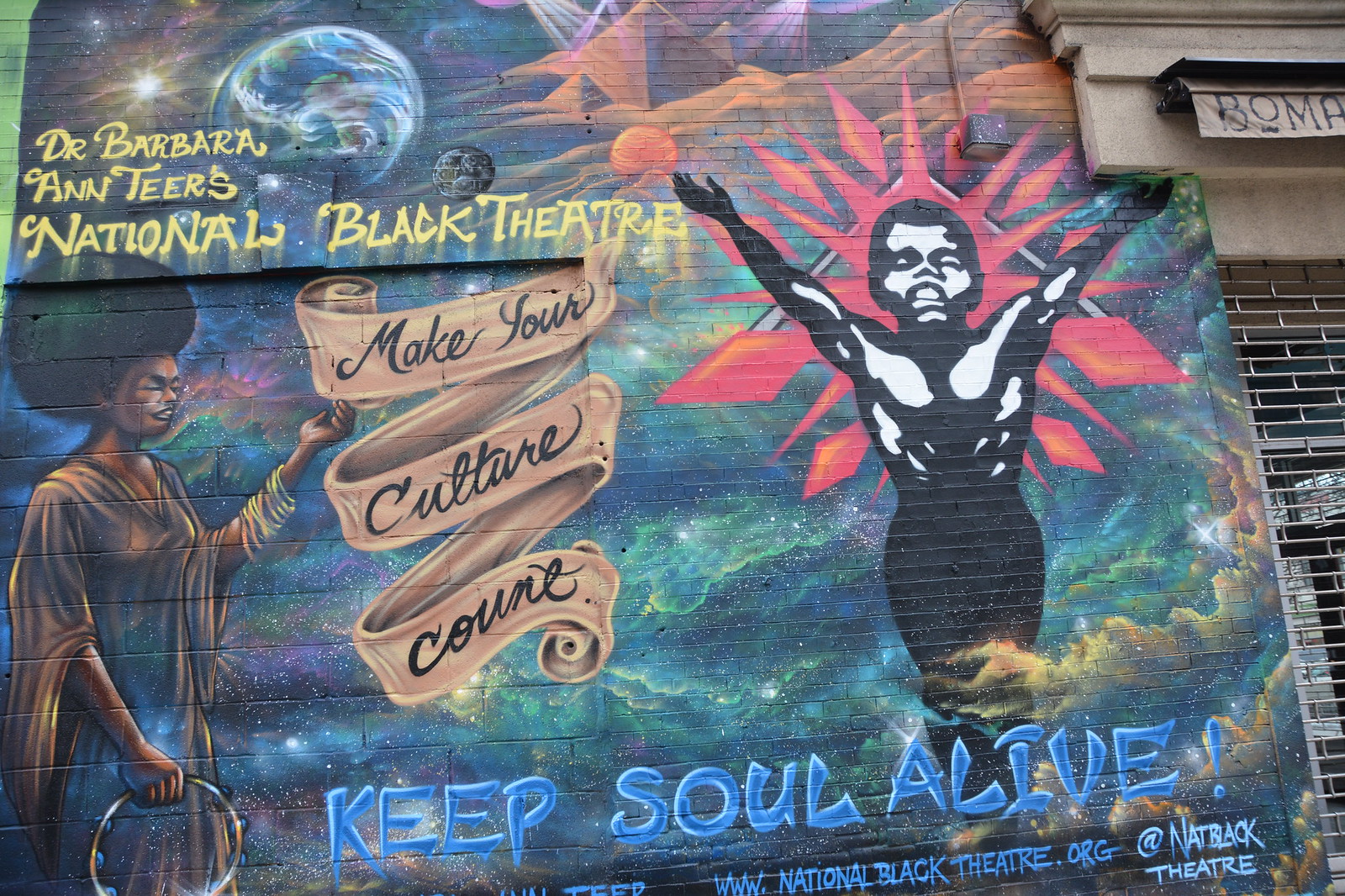The image showcases a vibrant mural painted on a brick wall, decorated with a mix of cosmic and cultural elements. At the top center of the mural, a depiction of the sun and a planet resembling Earth is featured, set against a backdrop of a blue, starry sky interspersed with clouds. Flanking the Earth are additional planetary images, resembling Jupiter or Saturn, creating a celestial theme.

Below this astral scene, pyramids rise from the desert sands, their sharp geometrical shapes adding to the mural's complexity. Prominently, a banner scroll, featuring the text "Dr. Barbara Ann Teer's National Black Theater," is emblazoned in yellow at the upper left corner of the mural. The mural's background transitions through various shades of green and blue, providing a lush setting.

To the left side of the mural, a black woman with a large afro and flowing gown holds a tambourine, her eyes serenely closed. This figure is positioned near the slogan "Make Your Culture Count," written on a scrolling brown ribbon. Over to the right side of the mural, an abstract image of a young black boy, depicted in dynamic motion with outstretched arms, appears to soar from a pyramid-like structure. Red, triangular rays emanate from behind him, enhancing the image's sense of energy and movement.

Towards the bottom of the mural, the words "Keep Soul Alive" are written in blue text, alongside the website "www.nationalblacktheater.org" and "at Nat Black Theater." Adjacent to the mural, metal railings and a gated entryway hint at the mural's urban setting. The awning above this entryway displays the text "B-O-M-A," adding another layer of context to the location of this intricately detailed artwork.